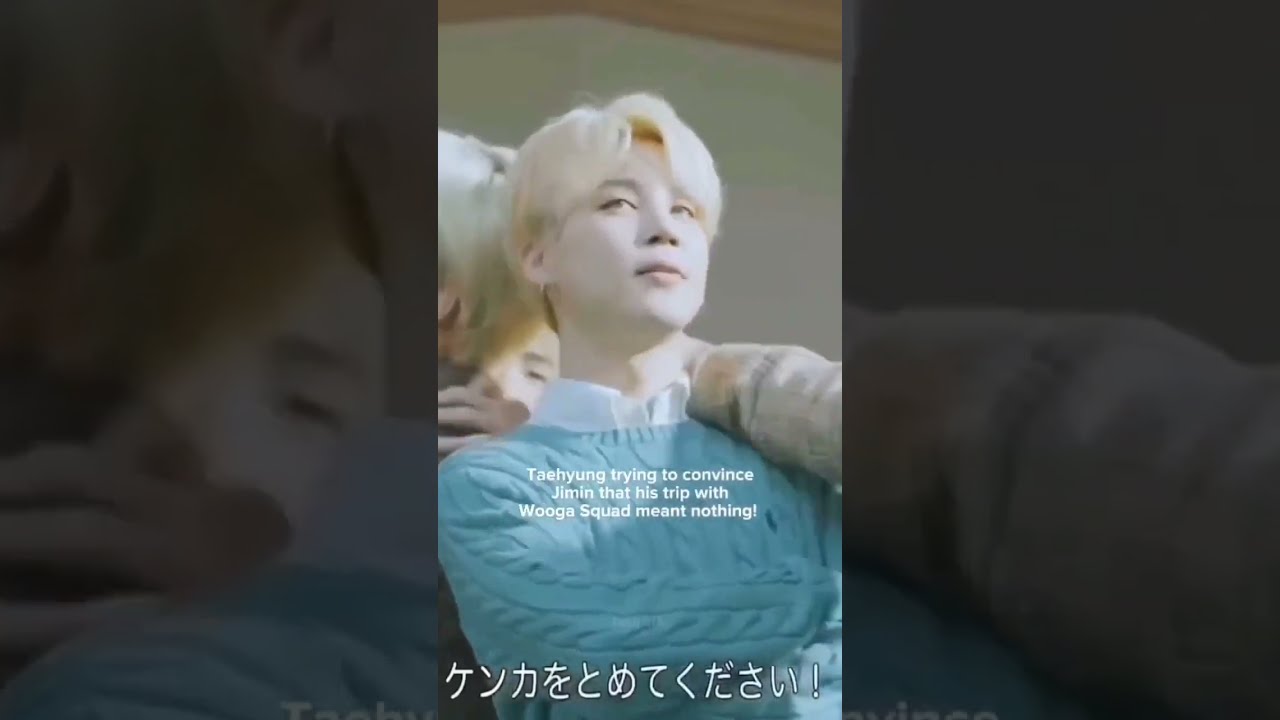The image depicts a striking portrait of a youthful, androgynous character with bleach blonde hair that is parted and swooping slightly over the forehead. The individual has extremely pale skin, almost giving an ethereal or artificially lightened appearance, and possesses delicate, feminine facial features that may make it challenging to discern gender at first glance. This character is facing forward, with a subtle tilt to the right and their gaze wistfully directed towards the upper left side of the frame.

They are attired in a light blue cable-knit sweater, with noticeable braiding down the sleeves, over a white button-down shirt with the collar peeking out. One hand is placed across their chest while the other is raised towards the shoulder. Additionally, another figure whose hair is similarly dyed blonde is partially visible behind them, adding to the overall composition.

The background of the picture features grey, blurred bars on both the left and right sides, suggesting the image might be a screenshot. Overlaying the image, towards the lower center, there are small white letters that read: "Taehyung trying to convince Jimin that his trip with the Wooga Squad meant nothing." Below this text, near the bottom of the image, is an Asian script with an exclamation point, though it's unclear whether it is in Chinese, Japanese, or Korean.